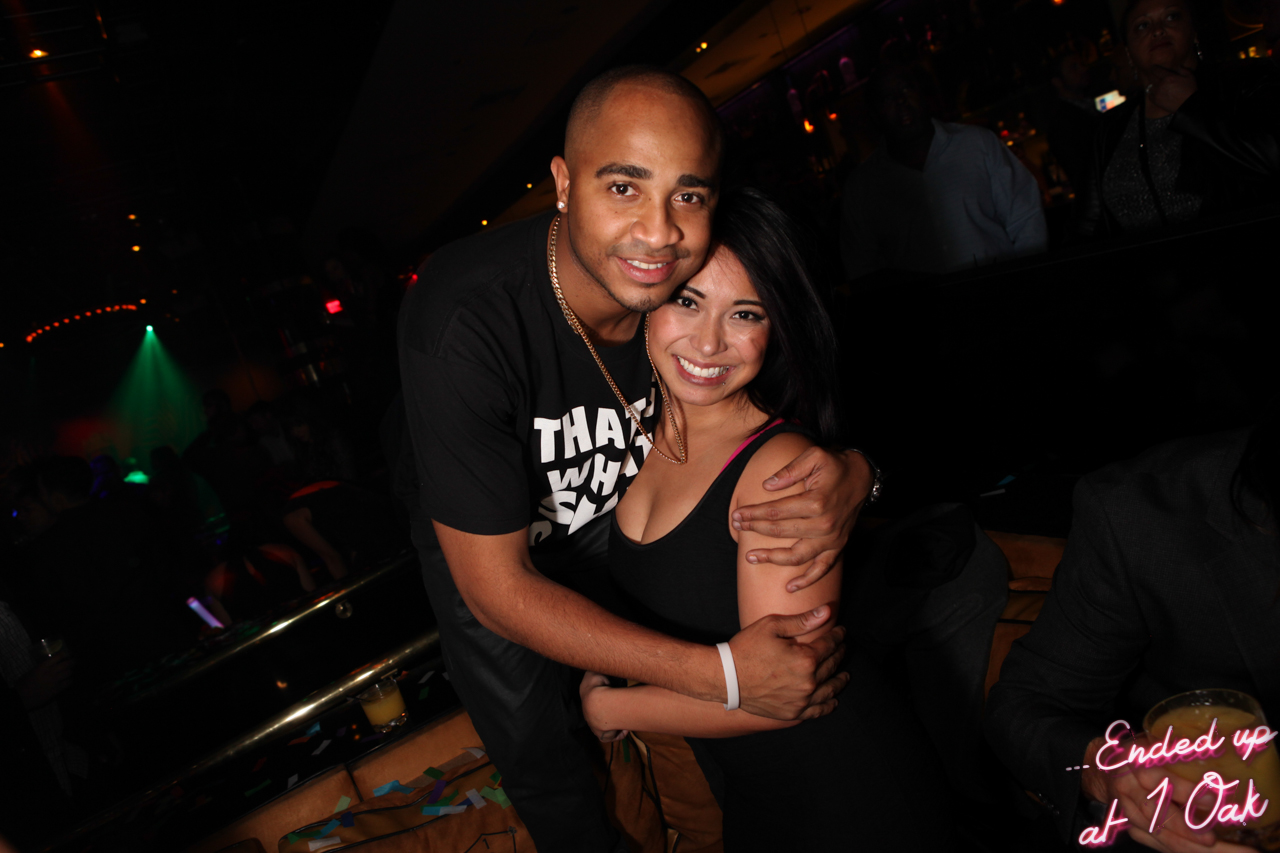In this photograph, we see a couple embracing inside a dimly-lit club or party hall. The setting appears lively, with some people dancing and engaging in activities in the background. The male is bald with light brown skin, dark eyes and eyebrows, and he is wearing a black t-shirt featuring white text along with black pants. A golden chain hangs around his neck, and his arms are wrapped around the woman. She has long black hair and is wearing a low-cut black dress. Both individuals are smiling warmly. Around them, various colored lights, including green laser lights, cast an ambiance over the scene. In the bottom right corner of the image, pink text reads "ended up at one oak," adding context to the location. There's a railing visible behind them, suggesting the photograph might have been taken on an upper level of the venue.